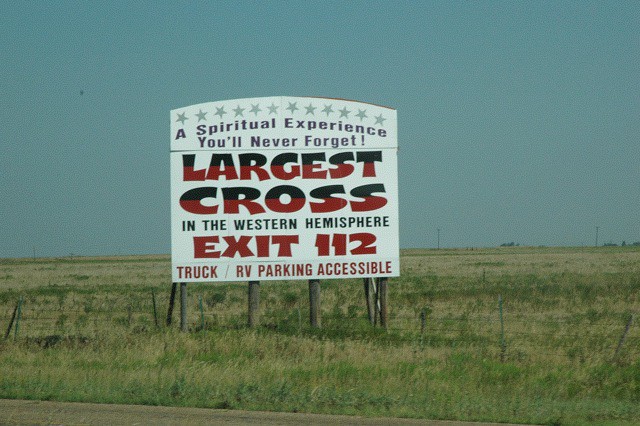In this image, a vast open field stretches out, covered in green grass. Dominating the scene is a large, white billboard held up by four sturdy wooden posts firmly embedded into the ground. The billboard features a striking design with twelve stars arranged in a row across its top edge. Bold red and black text on the sign promotes a notable attraction, reading: "A spiritual experience you'll never forget. Largest cross in the Western Hemisphere. Exit 112. Truck/RV parking accessible." The sky overhead is a clear, vivid blue, adding a serene backdrop to the prominent advertising display.